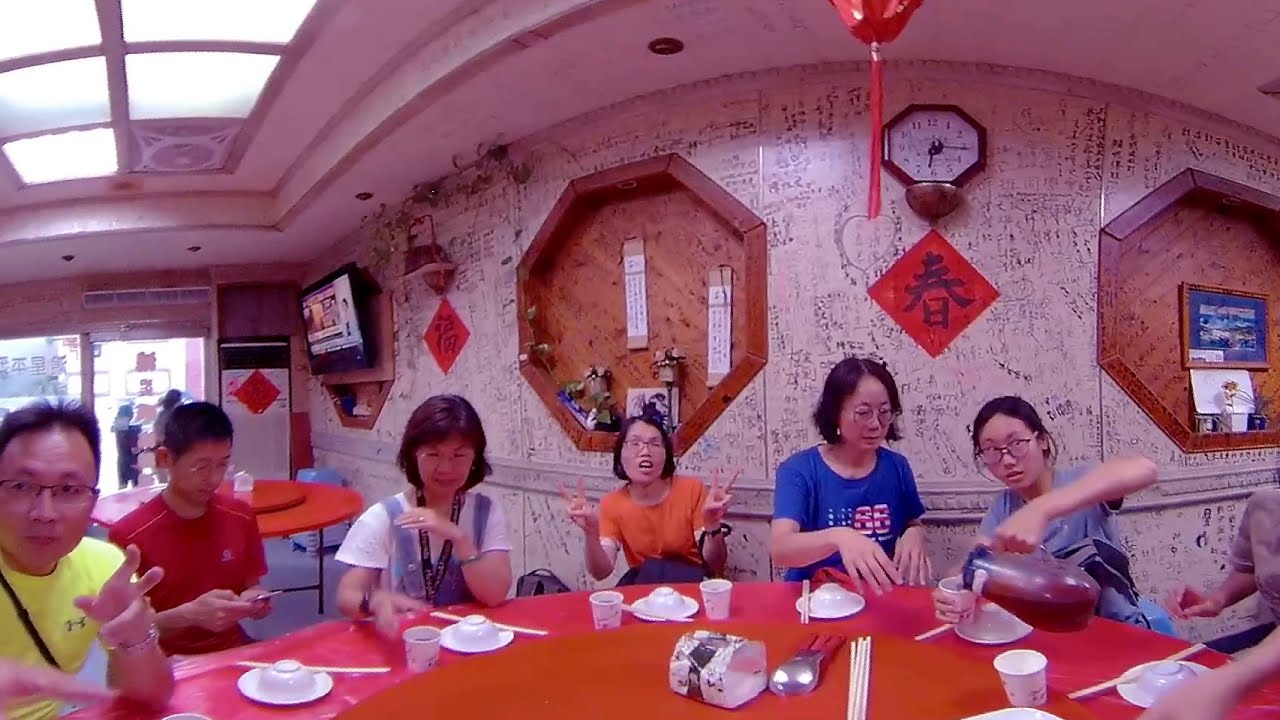A vibrant dining scene unfolds within a bustling Asian restaurant, likely Chinese, where a large round table with an orangish-red surface anchors the room. Seated around this table are seven individuals, likely of Asian descent, dressed casually in t-shirts. The table setting includes white plates each topped with an inverted bowl or cup, alongside neatly arranged chopsticks. An aura of conviviality pervades the air as one woman, positioned centrally and wearing an orange shirt, playfully flashes a double peace sign toward the camera. Beside her, another woman is pouring a drink. To the left, a man in a yellow shirt and a young boy absorbed in his phone add to the lively ambiance.

The restaurant's decor further enhances the cultural atmosphere. The walls behind the diners are adorned with handwritten Chinese characters and diamond-shaped signs. A clock showing 6:15 and a TV broadcasting something in the corner add modern touches to the traditional setting. Light streams through a door on the left, suggesting a sunny day outside, while pinkish lighting illuminates the interior. A sense of community and heritage fills the space, as if the walls themselves have stories to tell from countless gatherings.